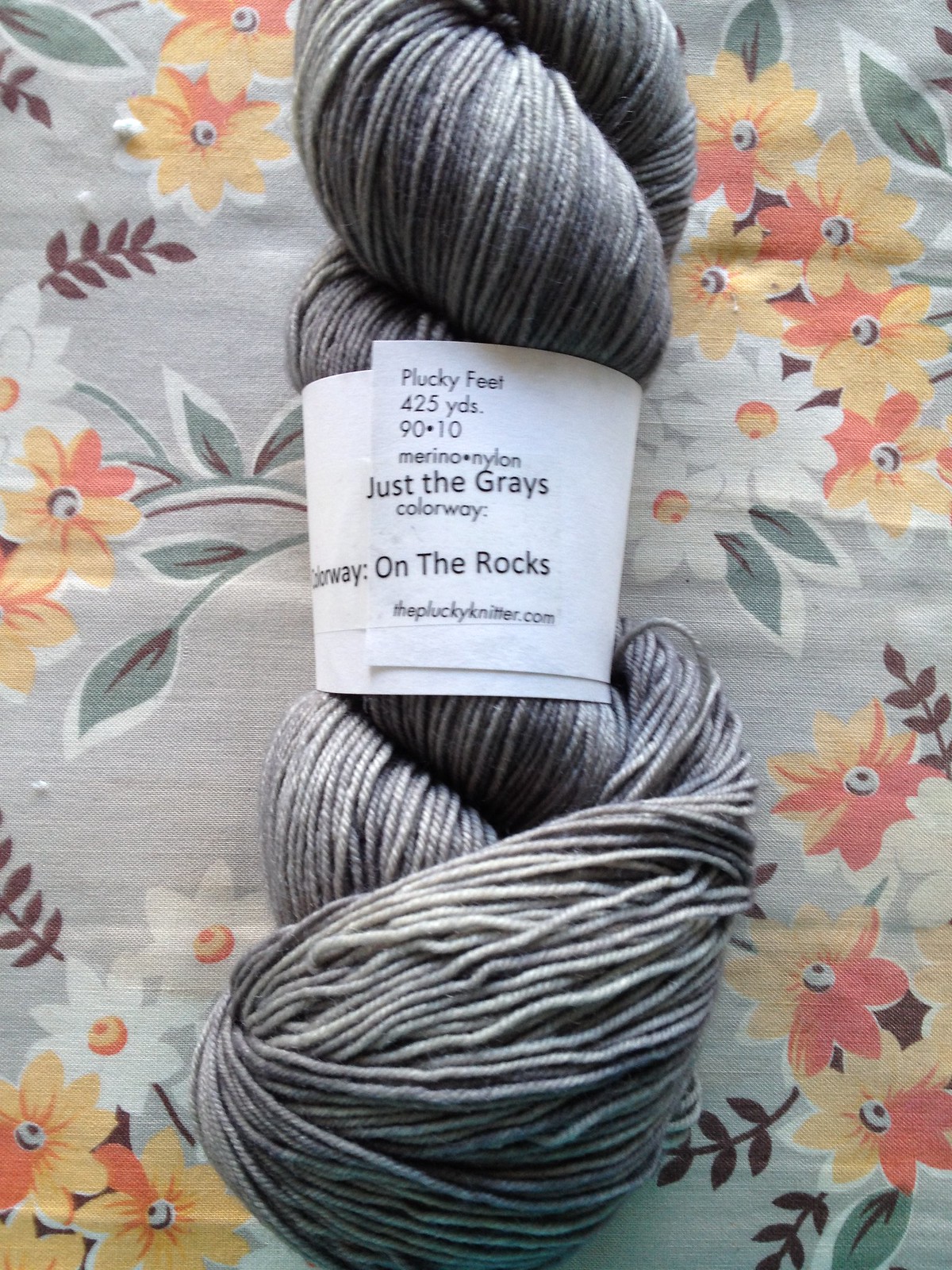The photograph is a high-resolution, horizontally rectangular image showcasing a skein of medium gray yarn with subtle variations in color. The yarn is twisted tightly and sits on a floral-patterned cloth, with no border framing the image. The focus is on the yarn, specifically its label, which is prominently wrapped around it. The label displays the brand name "Plucky Feet" and details such as "425 yards, 90-10 merino-nylon" blend. It also mentions the collection "Just the Grays" and the specific colorway called "On the Rocks." The label notes the website "thepluckyknitter.com," indicating the yarn is likely produced by a small, independent creator or company. The image is designed to highlight the color and texture of the yarn for potential customers.